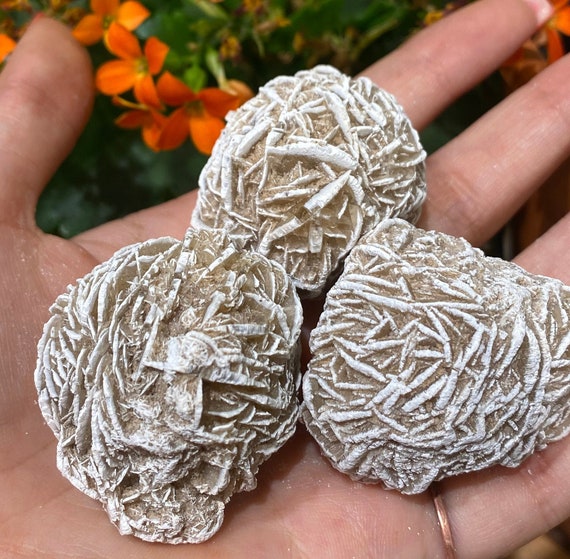In this detailed photograph, an outstretched left hand, adorned with a simple copper-colored wedding band on the ring finger, holds three intriguing rocks. The hand, likely belonging to someone of Caucasian descent based on its light pink hue, presents these irregular, grooves-ridden rocks, primarily light gray-brown but with striking white elements interspersed. These objects, reminiscent of fossils with potential plant imprints, captivate the viewer's curiosity about their origin. The backdrop reveals a green bush adorned with a vibrant orange flower, featuring three prominent petals, suggesting a setting of natural beauty. The snapshot, taken in daylight, leaves the viewer pondering if the rocks were collected during a vacation or part of a local exploration.